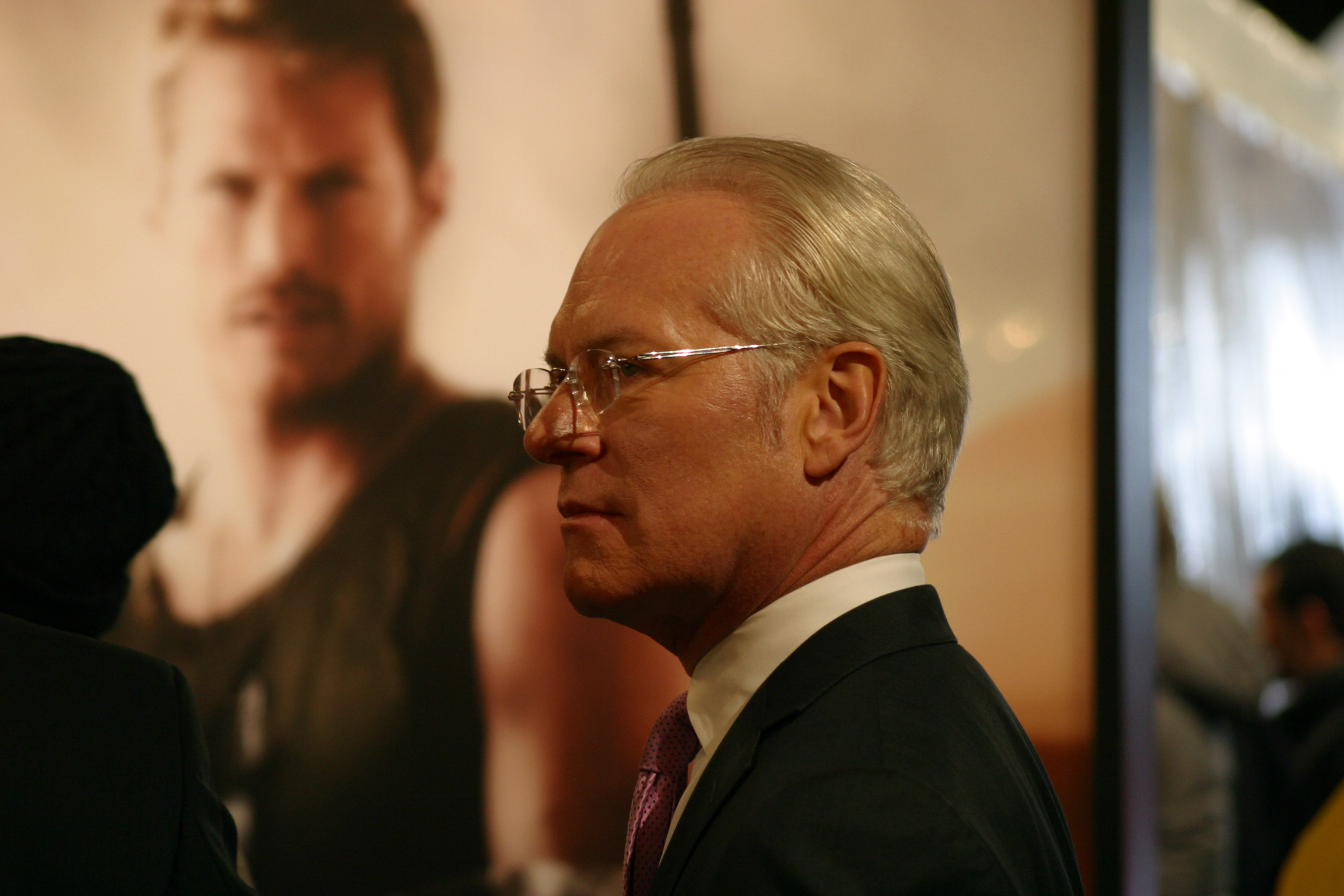The image features an elderly white male in the foreground, positioned towards the left, showcasing a side profile. He has slicked-back white and grey hair that is slightly receding, and he wears thin, silver-framed glasses that sit a bit down on his nose. His expression is serious, and he is dressed in a black suit jacket, a white collared button-down shirt, and a reddish-pink tie adorned with black dots.

In the background, partially out of focus, is a poster displaying a well-built male model with short brown hair, a noticeable mustache, and a beard. The model is wearing a brown tank top and looks straight ahead with a serious expression. Additionally, on the left side of the image, there is a figure in a darker suit, partially visible, while the right lower corner of the picture reveals another blurry figure, furthering the depth and complexity of the scene.